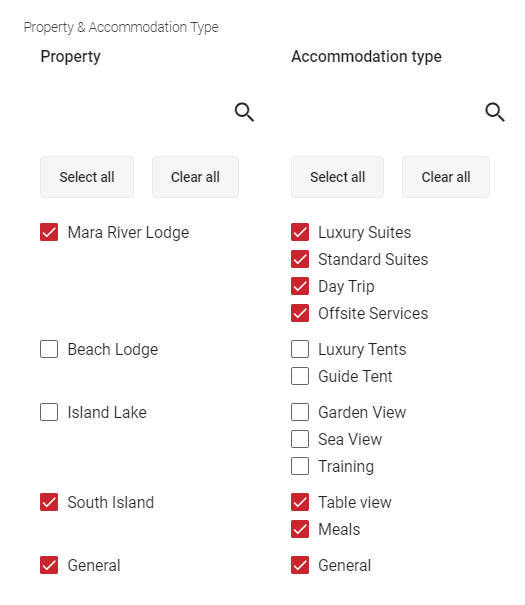The image displays a user interface for selecting various properties and accommodation types for a booking or search system. On the left side, there is a section labeled "Property" with a list of options including Mara River Lodge, Beach Lodge, Island Lake, South Island, and General. On the right side, there is a section labeled "Accommodation Type" featuring options such as luxury suites, standard suites, day trip, offsite services, luxury tents, guide tent, garden view, sea view, training, table view, meals, and general.

Each option can be selected or deselected using checkboxes. The interface includes buttons for "Select All," "Clear All," and a "Search" bar at the top, applicable to both sections. Currently, Mara Lodge, Mara River Lodge, South Island, and General under "Property" are checked off in red boxes with white check marks. Similarly, under "Accommodation Type," options selected with red boxes and white check marks include luxury suites, standard suites, day trip, offsite services, table view, meals, and general.

The background of the interface is white and features no icons or images, relying solely on text for making selections.